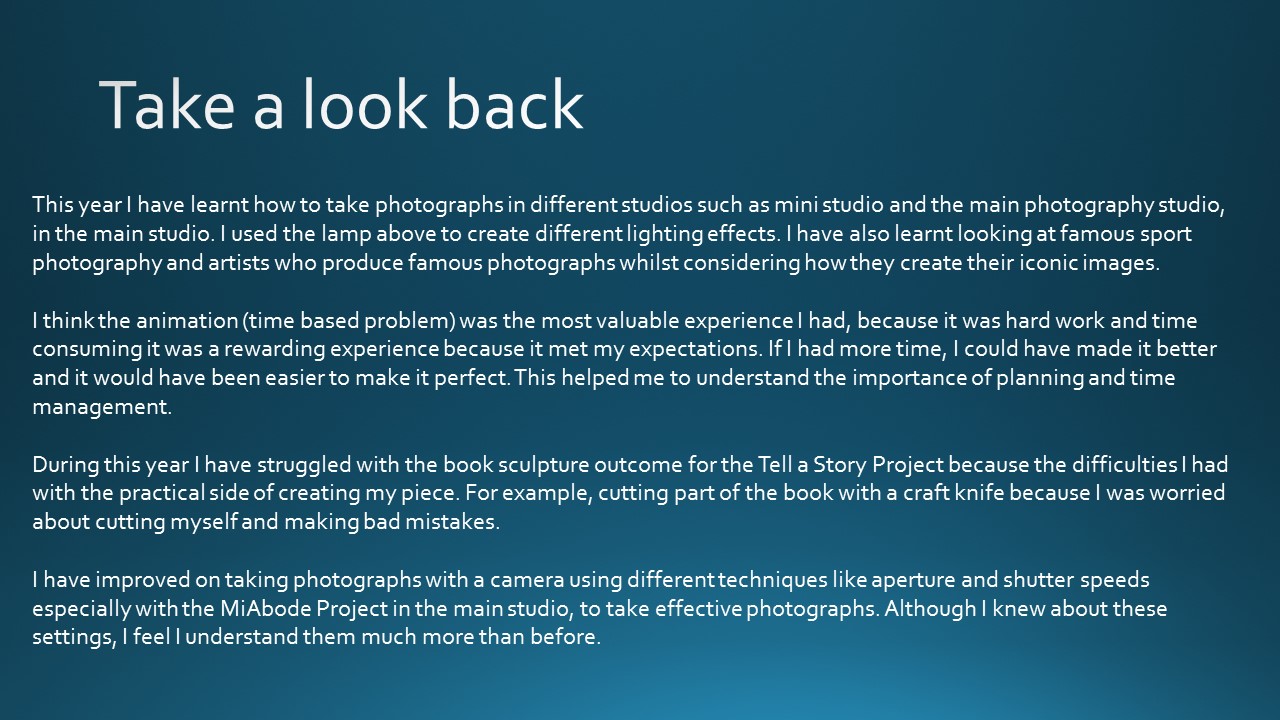This image features a predominantly blue background with white text, where the color gradient transitions from a lighter shade at the bottom to a darker shade at the top and along the sides. The heading, "Take a Look Back," is positioned at the top left of the image. The main content consists of four paragraphs detailing a reflective narrative. 

The text recounts the author's learning journey over the past year, starting with their experience in various photography studios, including a mini studio and the main photography studio. In the main studio, they experimented with lighting effects using an overhead lamp. The author also delved into famous sports photography and artists, analyzing how they create iconic images.

A significant part of their experience was the "Animation Time-Based Problem," which, despite being challenging and time-consuming, proved to be highly rewarding and met their expectations. This project emphasized the importance of planning and time management.

Another project, the "Tell a Story" book sculpture, presented practical challenges like using a craft knife, which caused concerns about safety and making errors. 

Throughout the year, the author improved their photography skills, particularly in using camera settings like aperture and shutter speeds, enhanced through the “My Adobe” project in the main studio. Although they were familiar with these settings, they gained a deeper understanding of their applications.

The detailed reflection underscores the author's growth and the various aspects of learning, skill development, and overcoming practical difficulties throughout the year.